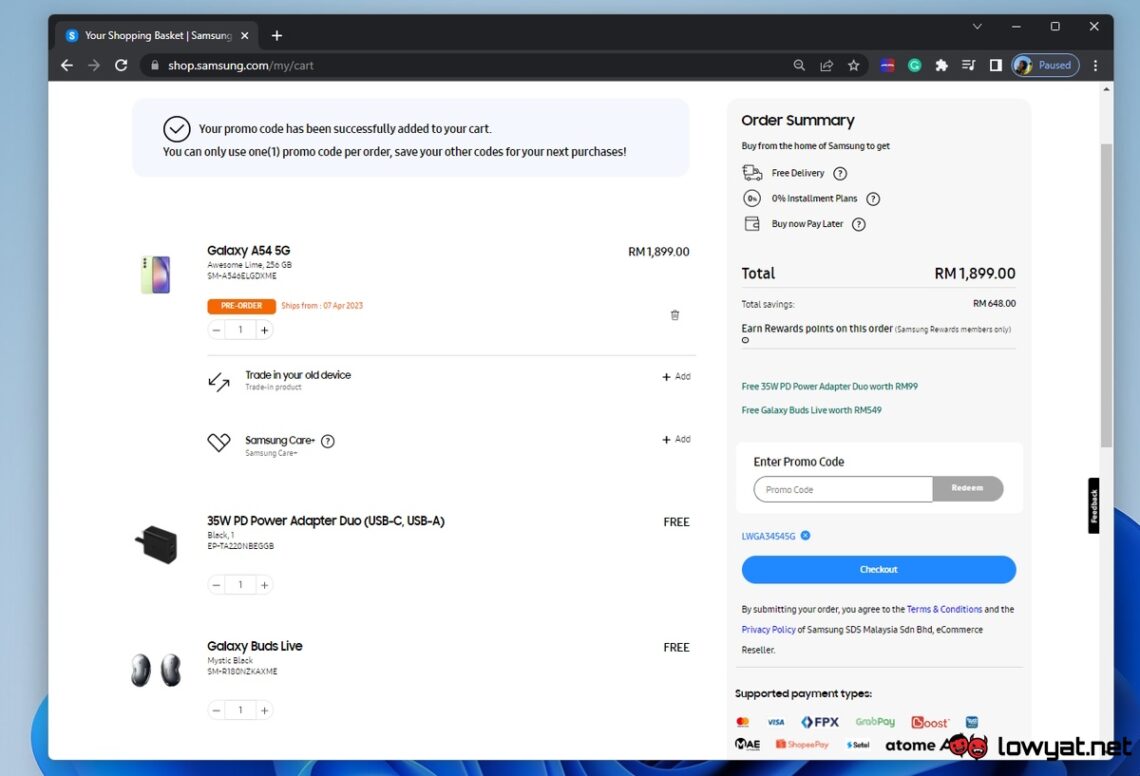The image displays the shopping cart on the Samsung website. In the cart, there's a Samsung Galaxy A54 5G smartphone priced at $1,899.00. No trade-in device has been added and Samsung Care has not been opted for. The customer has applied a promo code, which entitles them to two free items: a 35W PD Power Adapter Duo compatible with USB-C and USB-A, and a pair of Galaxy Buds Live. The order summary indicates a total of $1,899.00, with savings of $648.00 due to the promotion. To complete the purchase, the user simply needs to click the blue checkout button.